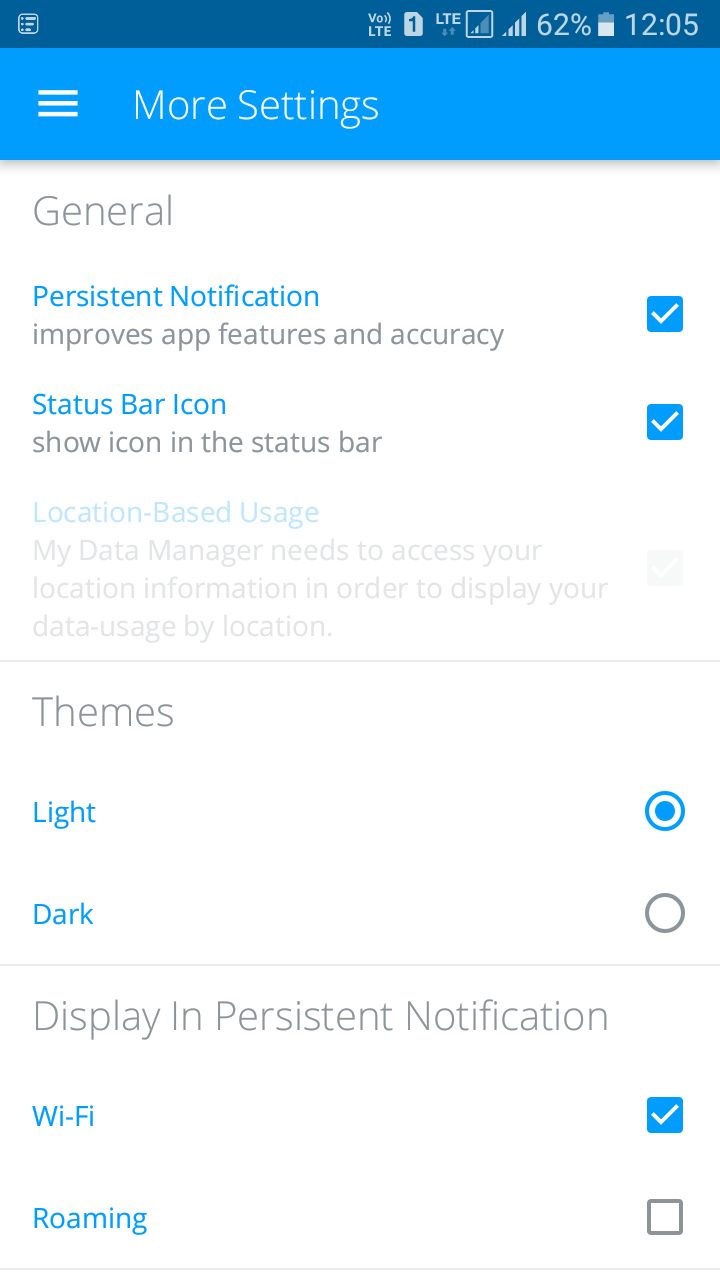This image is a screenshot of a cellphone's settings tab. At the top, there is a blue header labeled "More Settings" in white font. To the right of this text, there is a menu icon. The main body of the settings page has a white background. 

On the top left of the page, "General" is prominently displayed in large gray letters. Below this header, there is an option labeled "Persistent Notification," accompanied by a checkbox on the far right that is selected.

The next item down is "Status Bar Icon," which also has a checkbox to the right that is selected. 

Following this, the "Location-Based Usage" option is listed, but it is grayed out and its checkbox on the right is not selected.

Further down, a section is labeled "Themes" in large gray font. Under this category, there are two options: "Light" and "Dark." To the right of these options, there are radio buttons, with "Light" selected.

At the very bottom of the page, another category titled "Display" features options for "Persistent Notification." Under this, "Wi-Fi" is listed as the top choice with its checkbox selected. The option "Roaming" is below that and its checkbox is not selected.